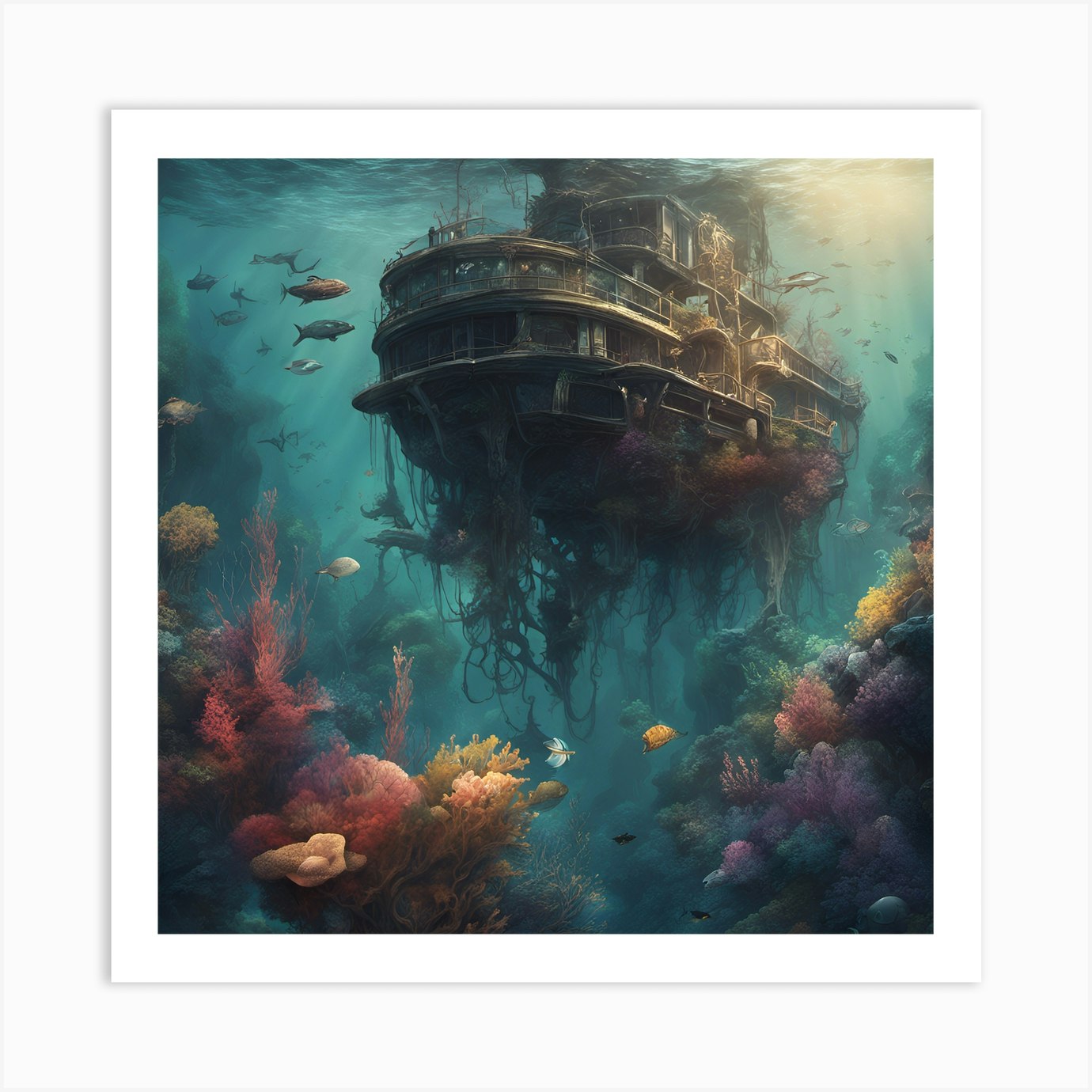The artwork is a vertically rectangular, full-color painting set within a dual border. The outer border is thick and off-white, while the inner border is thinner and bright white, creating a framed effect. The scene depicted is underwater, portraying a mesmerizing shipwreck. The ship itself is large, at least three to four stories high, and is mostly submerged, with just a small portion visible near the surface. The ship appears ancient and haunted, rotting away, adorned with barnacles, vines, and plant roots hanging from its underside. Surrounding the ship is a vibrant underwater ecosystem teeming with colorful life; various corals and plants in hues of pink, purple, yellow, orange, red, and green are interspersed with rocks and schools of fish swimming against the backdrop of blue water. Sunlight pierces through the surface from the upper right corner, illuminating the ghostly spectacle beneath. The overall image exudes a captivating and almost eerie beauty, showcasing the ruin and rebirth that takes place in the depths of the ocean.